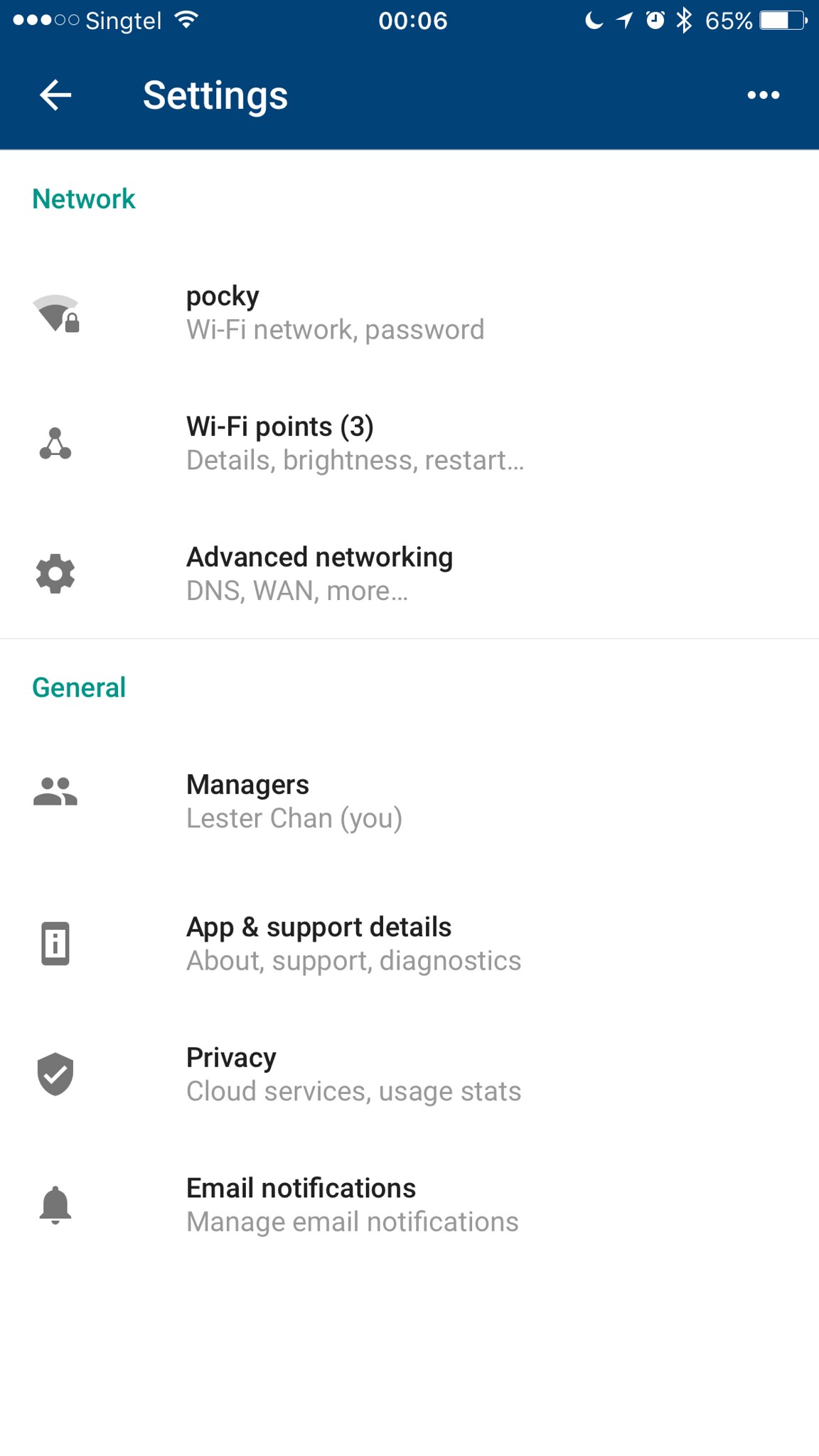The image captures a screenshot of a mobile phone's settings menu, specifically focused on network settings. At the top of the screen, the mobile carrier "SingTel" is displayed alongside the time, which reads 00:06, indicating it is late at night. Additional indicators show that the battery is at 65%, Bluetooth is enabled, and there is an active alarm set.

The section being viewed in the settings menu is titled "Network." The network name is "Parkey" and it also shows "Wi-Fi 3" and "Advanced Networking." Below this, there are several categories listed: "General," managed by "Lester Chan," labeled "You," and followed by options for "Apps," "Privacy," and "Email Notifications."

The top of the menu features a header with the word "Settings" and a back arrow, along with a three-dot menu for additional options. This header is presented in a royal blue color with white text. The sections for "Network" and "General" are highlighted in turquoise, while the remaining text is in varying shades of gray and black, adding a visually appealing contrast to the interface.